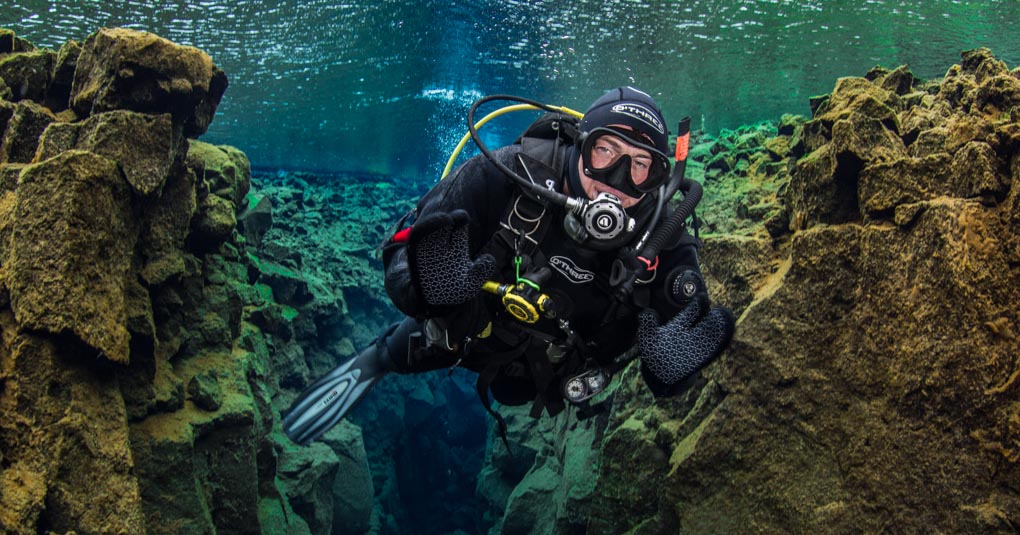In the image, an underwater photograph captures a male scuba diver clad in an all-black wetsuit, complete with a hood and gloves, prominently positioned in the center. His goggles are clear, revealing his light skin, and he breathes through a silver and black respirator with a black tube wrapping around to his back and a distinct yellow tube running down his back. His arms are extended towards the camera, palms up, displaying the light gray meshing on the undersides of his black gloves. Only one of his fins is visible trailing behind him.

The diver appears to be swimming upwards, possibly waving, amidst a strikingly clear and colorful aquatic environment. The water around him is a vibrant blend of green, turquoise, and blue, glistening with sunlight near the surface. Surrounding the diver is a dramatic rock formation consisting of brown stones, which transition to green further back, creating a cavernous effect. The diver hovers above a large crevice or canyon that extends downward below him. This vividly detailed underwater scene provides a mesmerizing glimpse of the scuba diver exploring the depths.